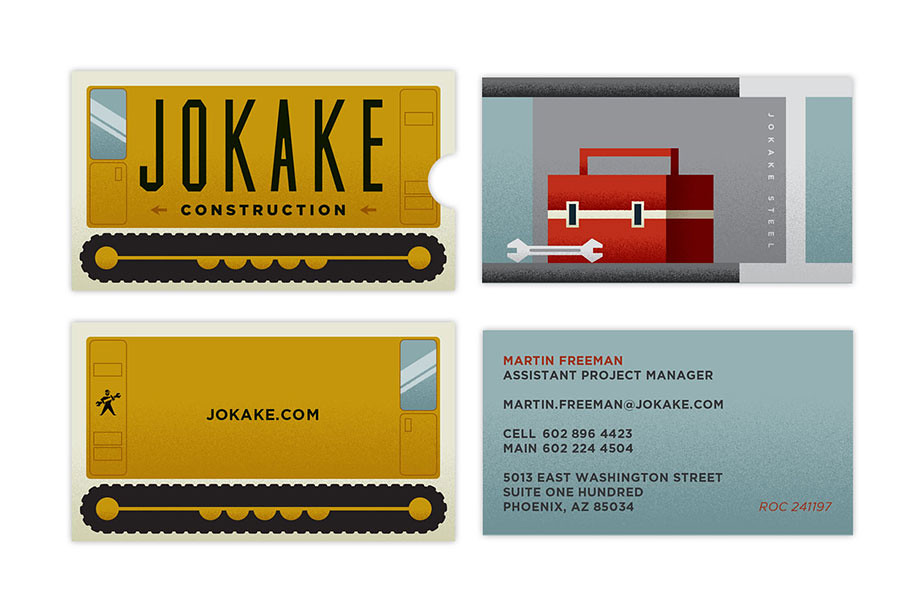This image showcases a detailed composite design for a business card presentation, featuring elements for both the front and back covers of a sleeve and the business card itself, laid out in a landscape orientation with four evenly divided sections. 

In the top left corner, the front cover of the sleeve displays a gold rectangle with the bold black lettering "J-O-K-A-K-E Construction." Underneath, a black horizontal strip mimics the tracks of heavy construction equipment, giving the illustration the appearance of a tractor viewed from the side. Directly beneath this image, the back cover of the sleeve mirrors the front but shows the back side of the tractor. 

To the right, the front of the business card includes a design with an aqua and gray color scheme, featuring a red toolbox overlaid with a white wrench. The back of the card, positioned at the bottom right, presents the name "Martin Freeman," his title "Assistant Project Manager," contact details including his email "Martin.Freeman@JOKAKE.com," and cell phone number, all set against a blue background with typography in red and black. The address "2013 East Washington Street, Suite 100, Phoenix, Arizona" is also included, showcasing a cohesive and professional design.